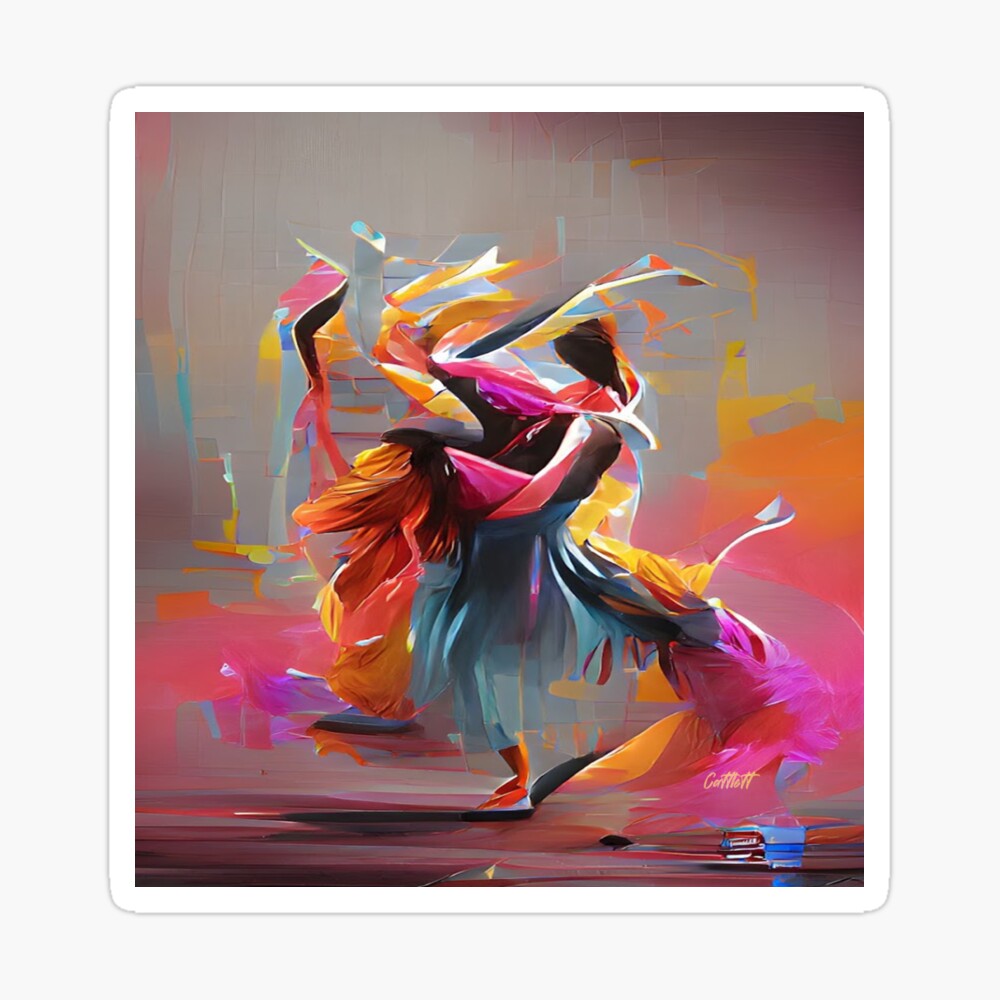This is an abstract painting, likely representing two dancers in graceful motion, their forms suggested by flowing geometric shapes and vibrant, dynamic colors. The central figures seem to intertwine, conveying the essence of dance, with recognizable elements such as feet, a head, and what might be a blue skirt or dress. The composition is filled with a spectrum of colors including yellow, orange, pink, lavender, light blue, red, black, brown, tan, and gray, blending seamlessly to create a sense of energy and motion. The background itself shifts through these hues, amplifying the feeling of continuous movement. In the lower right corner, there is a signature in yellow—perhaps the artist’s—though it is partially obscured and difficult to decipher. The painting is framed with a white border, set against a gray backdrop, enhancing its vibrant, almost poetic expression of light, energy, and grace.